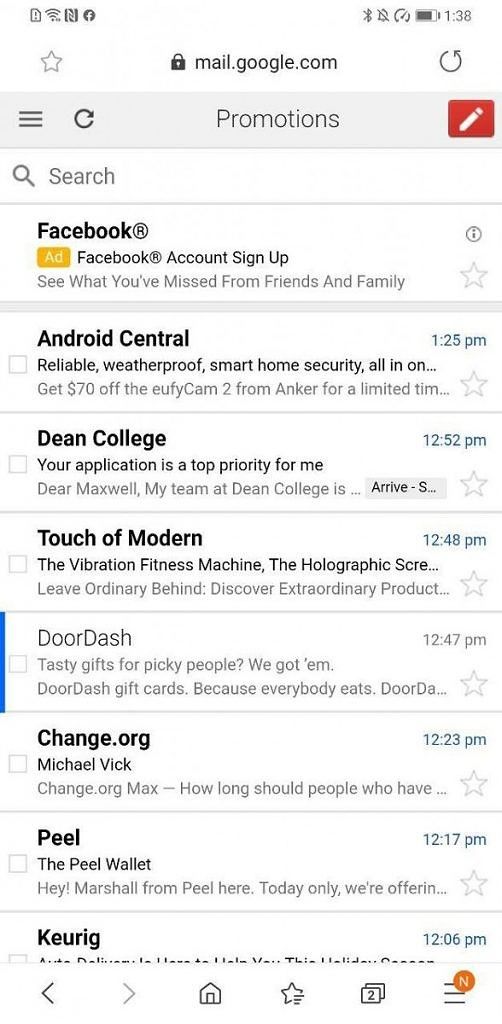The image displays a user's phone screen opened to the "Promotions" tab in the Gmail app. At the top of the screen, the status bar indicates a mostly full battery, the current time of 1:38, and silenced notifications. The secure connection icon along with "mail.google.com" is visible. On the left of this address, a star icon to favorite the page is present, followed by a refresh symbol.

Below the status bar, a light gray banner with the word "Promotions" in bold black text is centered. On the left of this banner are a refresh button and the three-horizontal-lines menu icon. To the right, there is a conspicuous red edit button.

In the main content area under the "Promotions" heading, multiple email promotions are listed on a white background. The promotions shown include emails from Facebook, Android Central, Dean College, Touch of Modern, and DoorDash, with DoorDash highlighted by a bright blue vertical stripe next to it, indicating selection. Additional promotions from Change.org, Peel, and Keurig are also visible.